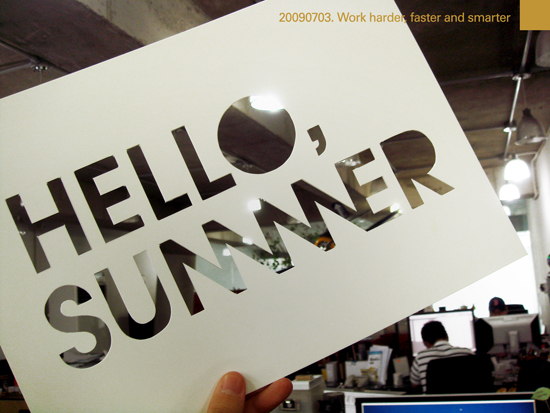In the center of the image, a hand is holding a horizontal, rectangular white card with the words "hello summer" in mirrored, gray letters. Above these words, in the top right corner of the card, the text "2009 07 03" is visible, followed by the motivational phrase "work harder, faster, and smarter." The card is prominently positioned in the middle of the image. In the background, which indicates an indoor, likely office setting, two people are seated at desks with computers. Various colors, including blue, white, black, green, yellow, orange, gray, and tan, are present in the scene. The floor and overhead lights are also visible, adding to the workspace atmosphere.